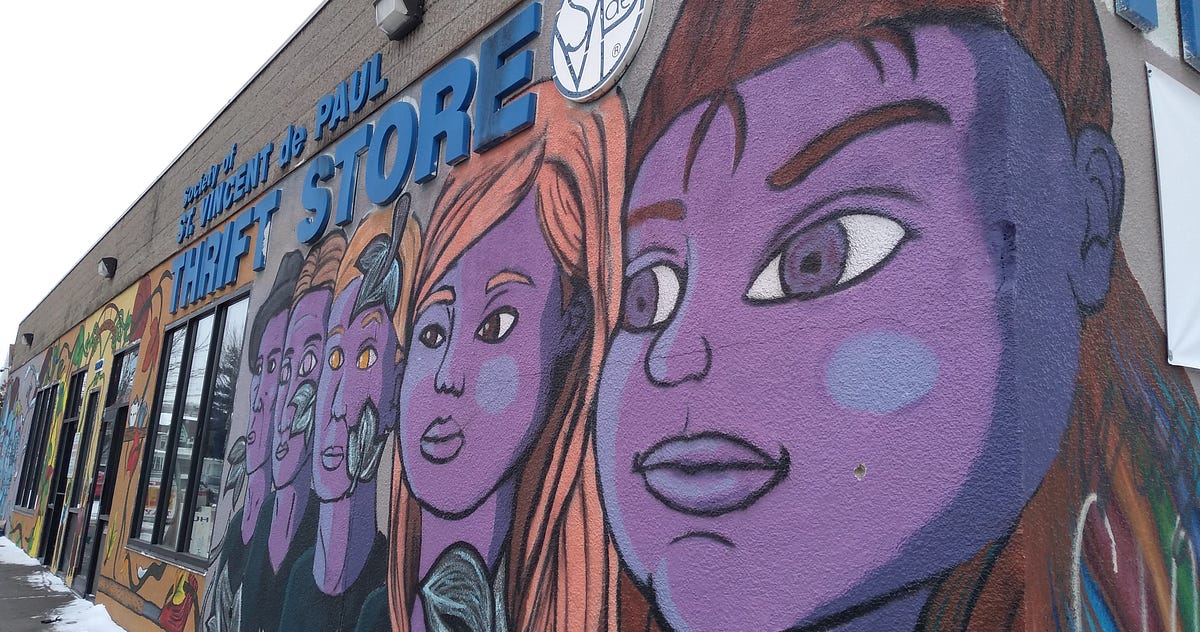In this image, we're viewing the side of the Society of St. Vincent de Paul Thrift Store, recognizable by its blue signage above the side of the building. The building's wall is adorned with an artful graffiti mural depicting a series of young faces with purple skin complexions and multicolored hair, a striking visual against the snowy backdrop. The mural begins with a plump little face with brown hair and eyelashes, followed by a young girl with blondish-reddish hair, and then a man with a hat. Beyond them are a couple more figures with hair ranging from orange to dark brown. Some of these faces feature artistic elements like black and white leaves. The mural leads up to the row of windows beside the front doors of the thrift shop.